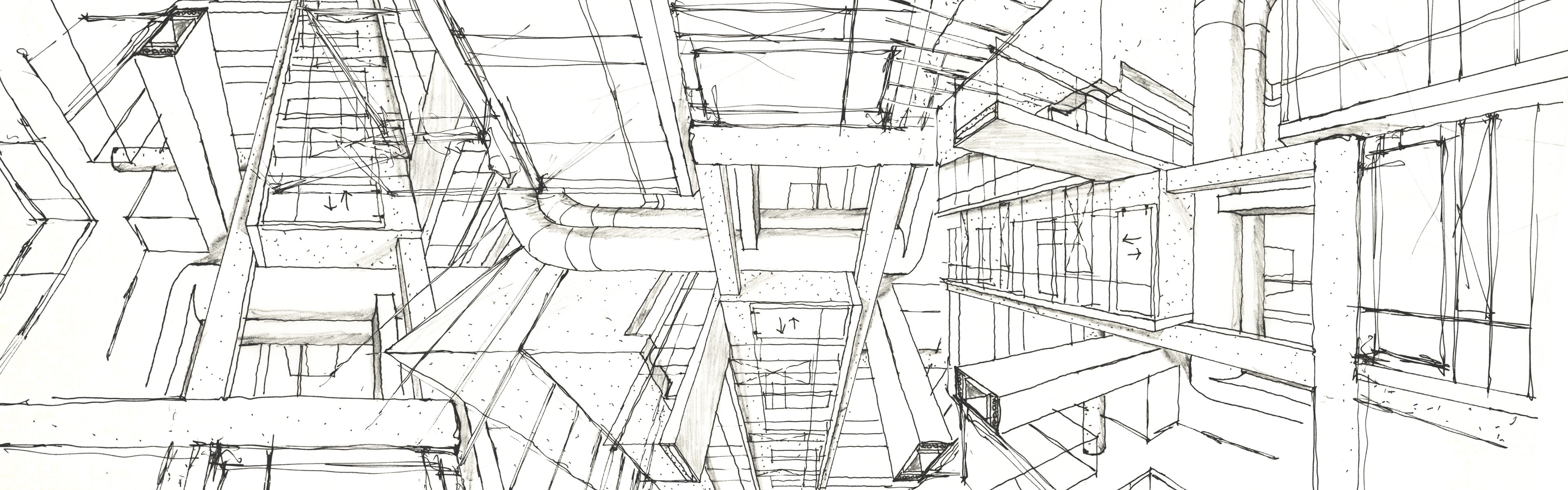The image showcases a detailed architectural line drawing on a white background, characterized by its long rectangular shape, approximately four times as long as it is tall. The black line work includes sketch-like lines, giving it a hand-drawn feel. The composition appears to present multiple perspectives of a structure, likely an architectural blueprint or model specs. The central focus seems to be an interior section of an unfinished building, possibly featuring beams, pipework, and an array of lines that suggest various structural elements like pipes, steel rods, or a shaft—potentially even an elevator shaft. There are arrows in the left, middle, and right thirds of the drawing which seem to indicate different viewpoints or directions, aiding in understanding the perspective from which these elements should be viewed. Overall, the drawing comprises a complex arrangement of shapes and lines, demonstrating a three-dimensional object through multiple angles, though the exact nature of the structure remains somewhat ambiguous.